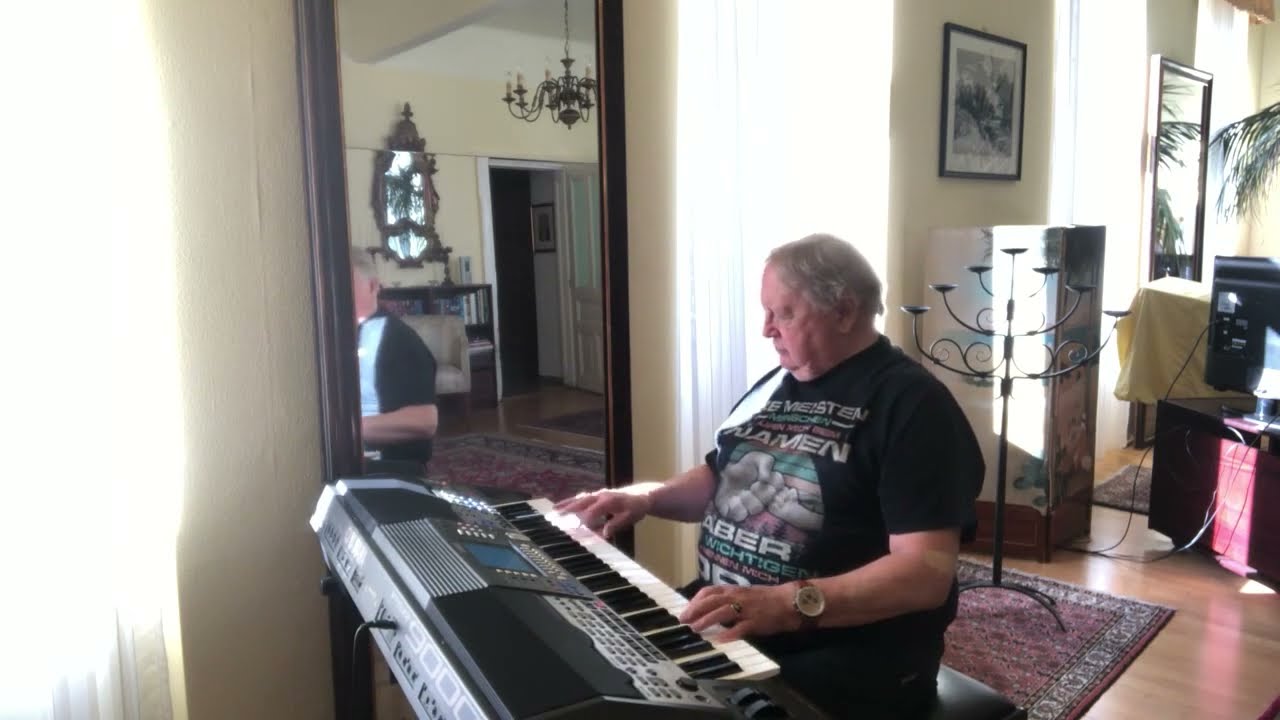In this detailed image, an older man with short, graying hair is seated at a keyboard, deeply engrossed in playing. He is dressed in a white graphic t-shirt with indistinguishable writing and sports a large watch and a ring on his left hand. The room appears to be a living area, its atmosphere set by the sunlight filtering through a window veiled by a curtain behind him. The wooden floor beneath is partially covered by a red rug, upon which a grand candelabra rests. To the side of the keyboard, a very tall mirror reflects parts of the room not directly in the photo, showcasing additional elements such as a chandelier, a television on a stand, a small dresser with a framed picture above it, and a door. The mirror also reveals a glimpse of the houseplant, likely a palm tree, to the right of the image. This well-lit room, featuring personal and decorative items like framed photos and a candle holder, creates an inviting backdrop for the man passionately playing his keyboard.